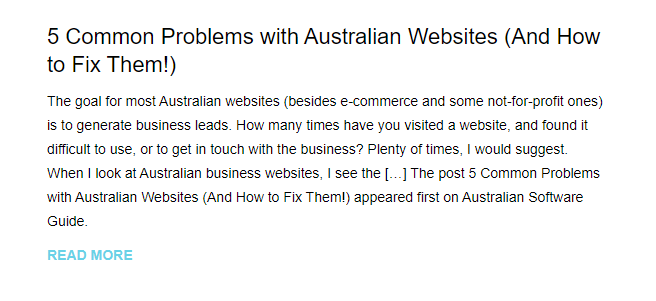**Image Caption:**

The image features a white background with black text that reads: "Five Common Problems with Australian Websites (and How to Fix Them)." This text is a headline designed to catch the reader's attention and highlight the main focus of the article. The primary aim of most Australian websites, excluding e-commerce and some not-for-profit ones, is to generate business leads. The text goes on to prompt readers to reflect on their own experiences with difficult-to-navigate websites, suggesting this is a common issue. The image includes a partial quote: "...the post Five Common Problems with Australian Websites (and How to Fix Them) appeared first on Australian Software Guide," indicating the source of the content. A blue "Read More" link is also present, encouraging further engagement with the article. The overall message in the image drives home the importance of addressing common website issues to improve functionality and lead generation.